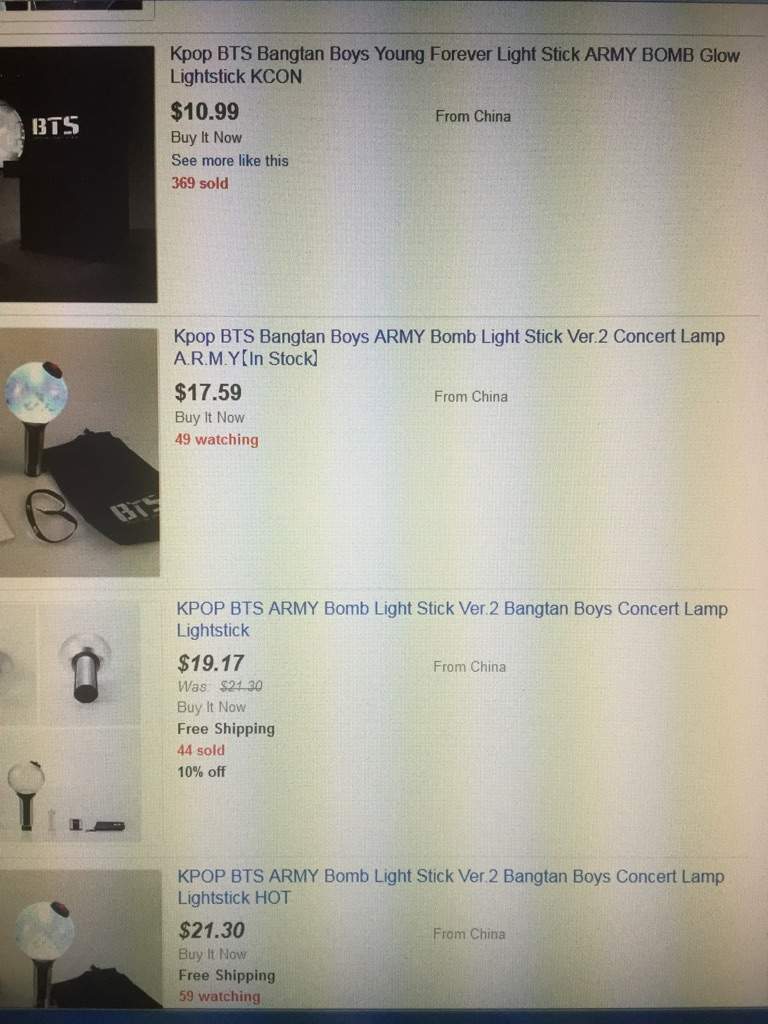A vertical rectangular image showcasing a list of search results, with the top result partially cut off. Along the left side of the image are black and white thumbnails of search results. The first visible thumbnail features the white letters "BTS" against a dark background, partially cropped. 

The second thumbnail appears on a gray background, depicting a small circular lamp with a hat-like shape on its right side and a black body, next to a black ribbon-like object and a small black bag with the gray letters "BTS."

The third thumbnail displays very light gray images: the left image is partially cut off, while the right one resembles a light bulb lying on its side, and another bulb standing upright underneath.

The fourth thumbnail resembles the second one, set against a darker gray background, featuring the same lamp-like object and black bag.

Accompanying each thumbnail on the right is a detailed description. The first item is labeled "KPOP BTS" in capital letters, followed by "Bangtan Boys, Young Forever, Light Stick," and "ARMY Bomb Glow" in all caps. Below the description, it states "Light Stick KCON," priced at "1095" in black text, "Buy It Now," and "See More Like This" in red font. Additionally, it notes "369 sold" and "From China" next to "1099."

The search results continue with similar details for each item, including the name, price, purchase options, number of items sold or watched, and origin from China.